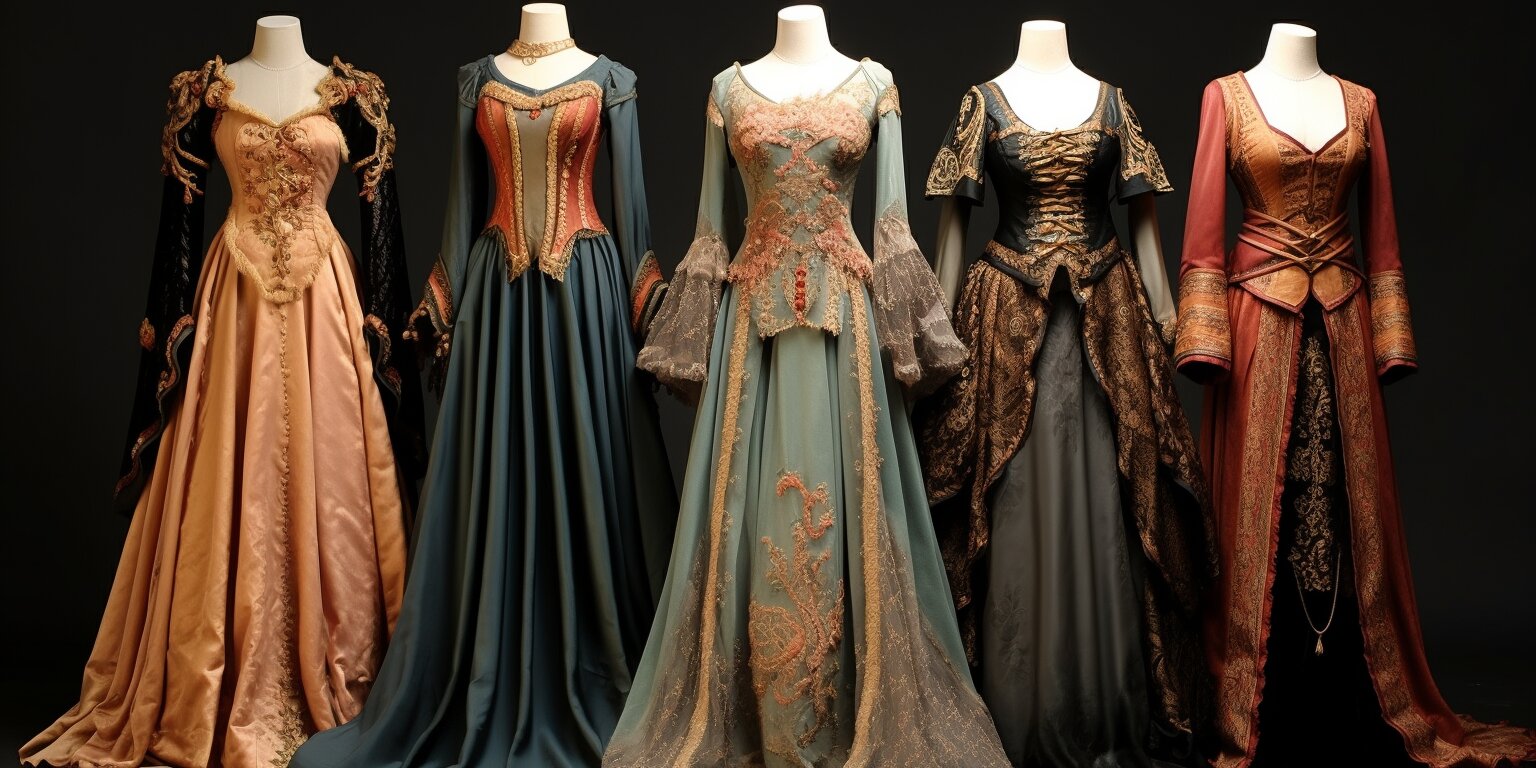The photograph showcases five headless mannequins modeling richly detailed, period-inspired gowns against a stark black background. Each dress is distinct and exhibits elaborate craftsmanship characteristic of medieval or renaissance styles. 

From left to right:
1. The first gown is a soft peach color with black, long sleeves adorned with intricate gold designs.
2. The second dress features a striking combination of turquoise blue and red with a grey middle, and its corseted bodice is framed by long, flowing sleeves and a layered skirt.
3. The central gown is a lighter seafoam green, highlighted with coral embellishments and flared long sleeves, exuding a whimsical charm.
4. Next, is a dark, deep blue dress with short sleeves and gold accents, including copper and gold embellishments on both the skirt and the bodice.
5. The final gown is an opulent red with gold patterns and a dramatic, opening skirt that reveals a contrasting black underskirt. 

All the dresses extend beyond the feet of the mannequins and exhibit intricate designs, rich colors, and flowing fabrics that evoke a sense of historical grandeur.